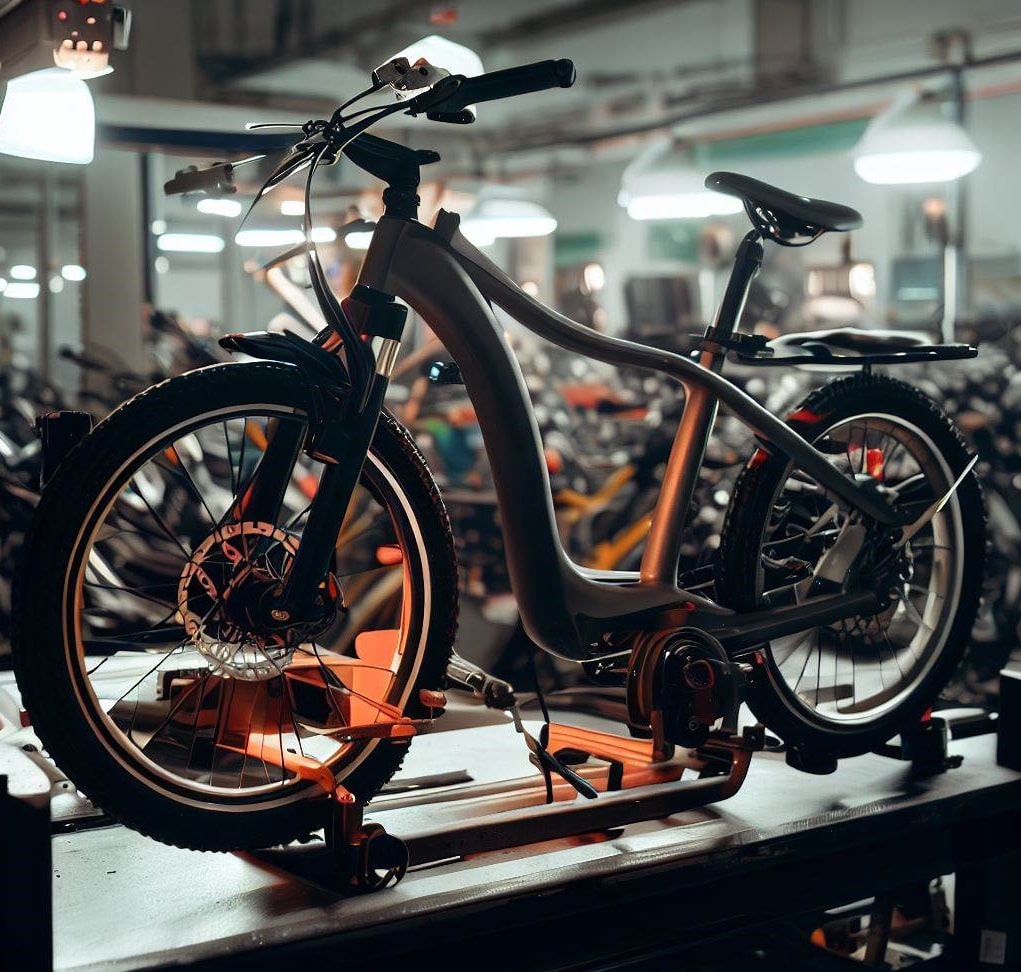The image depicts a bicycle mounted on a stand, prominently situated in what appears to be a large bicycle repair shop or possibly a small factory. The bicycle, shadowed and predominantly colored in blacks and grays, is being held by orange clamps on the wheels. It features a modern, slightly L-shaped frame design with a horizontal tube that supports the seat and a rear rack for carrying items. The bike has black, spoked wheels with notable orange and wavy artifacts around the spokes, suggesting it might be an AI-generated concept image. The front wheel is equipped with a brake disc, and the tires are thick, reminiscent of a hybrid between street and mountain bike tires. Despite some ambiguity about its nature, the bike appears to be a non-electric pedal bike. In the blurred background, several other bicycles can be seen, enhancing the busy atmosphere of the repair shop.